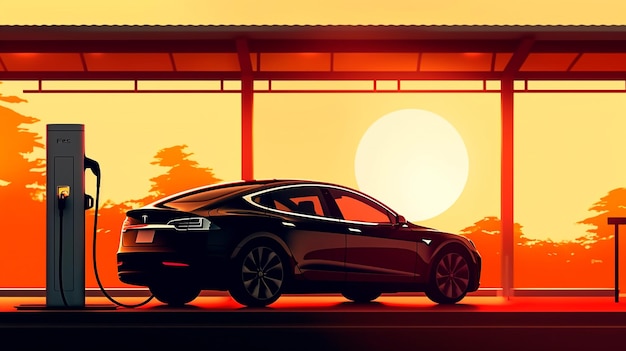In this digitally rendered image, a sleek, shiny Tesla saloon car is tethered to an electronic charger, with its distinctive logo visible on the rear. The car, meticulously illustrated with a digital felt-tip pen, showcases intricate wheel designs and has a polished, four-door exterior. Set against a backdrop of several trees painted in vibrant orange hues, the scene is illuminated by a low sun, casting a warm glow and suggesting either a sunrise or sunset. The surrounding architecture, reminiscent of traditional Japanese design, hints that the setting could possibly be somewhere in Japan.